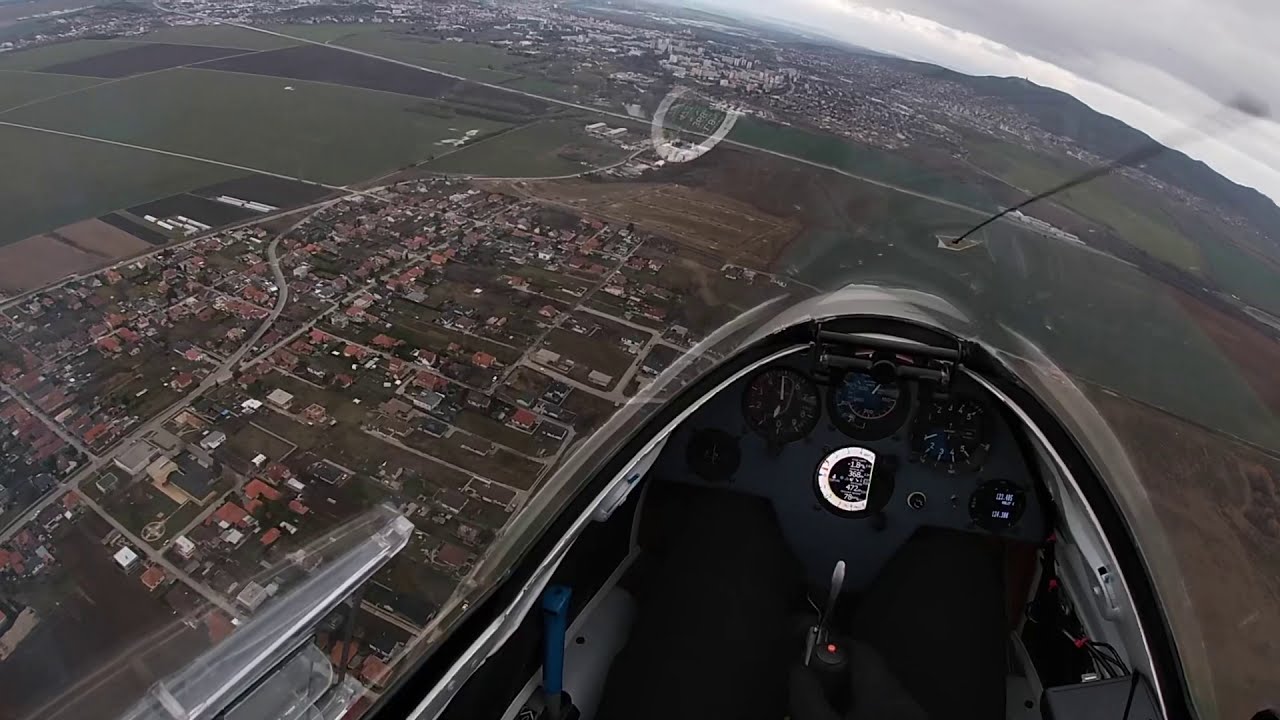This detailed aerial photograph is taken from within the cockpit of a glider, offering a front-seat perspective through a plexiglass canopy. The cockpit itself is simple and predominantly black, housing various instruments and gauges such as airspeed, altitude, and orientation indicators. A distinctive feature is a yoke, resembling a steering wheel but designed for aviation control, and a blue handle, likely for landing gear. Above the canopy, a faint, possibly distorted image of a cable or antenna is visible.

The view outside the cockpit reveals a sprawling landscape below, characterized by a mix of farmland, housing developments, and intersecting roads and interstates that weave through the scene. The colors are primarily green and brown, indicative of the lush farmland and urban areas, with additional dashes of white and red. Off in the distance, larger housing areas and mountainous terrain can be seen under a sky adorned with thick, varied cloud cover. Some clouds appear darker, suggesting imminent rain, while patches of blue sky peek through, adding depth to the horizon.